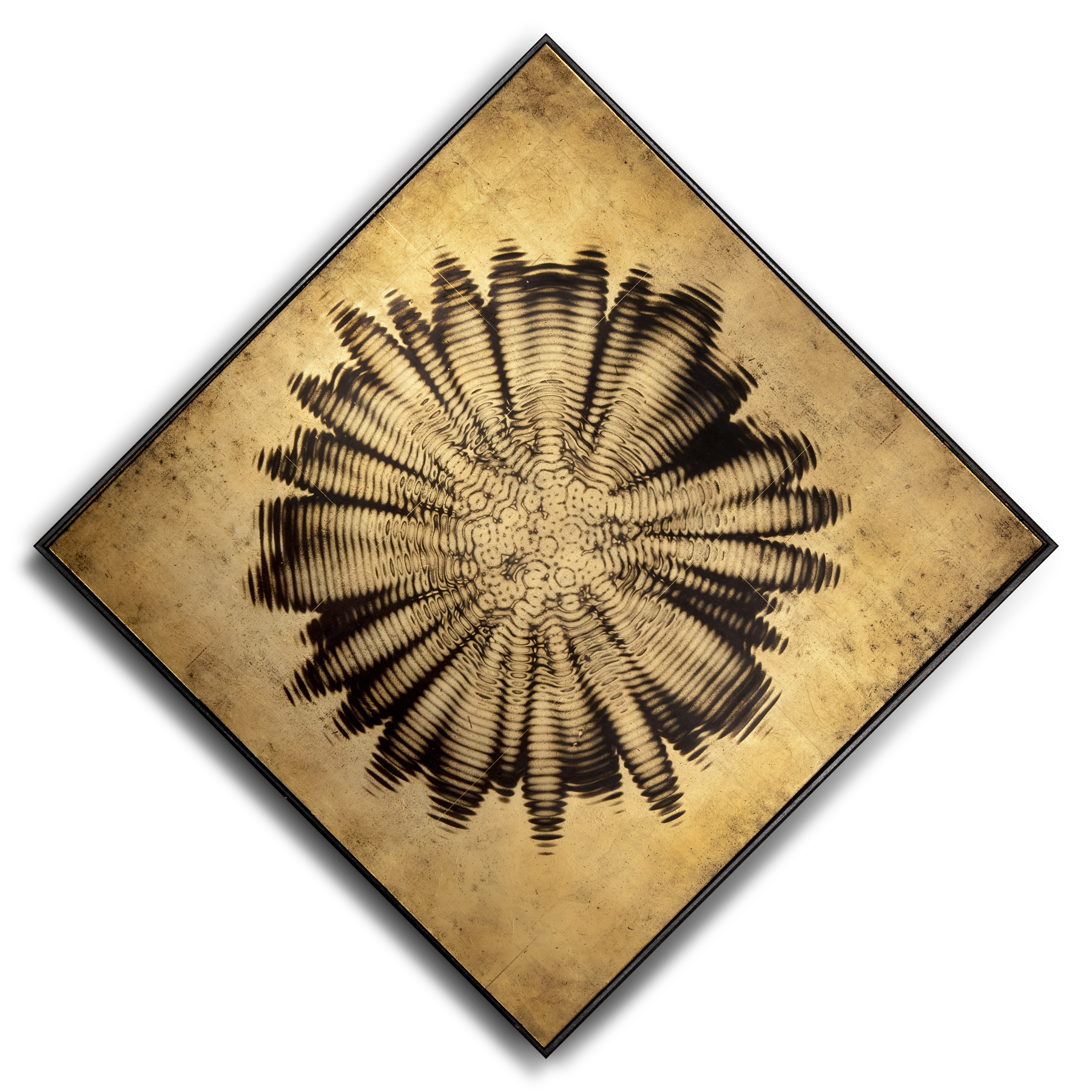The image depicts a square canvas rotated 45 degrees to form a diamond shape, giving the appearance of being centered on a light drop shadow. The canvas resembles parchment paper bordered with a thin black frame. Dominating the middle of the diamond is a complex, swirling vortex or radial design which appears dynamic and in motion. This intricate design resembles both a flower with numerous petals and radiating columns, characterized by thick and thin lines creating a dizzying, soundwave-like pattern. The coloration of the central design exhibits a blend of black, beige, and various shades of brown, with uneven hues and specks adding to the textured appearance. The entire artwork sits against a white background, highlighting its intricate details and contrasting colors. The piece suggests a rich, artistic quality, capturing the viewer's attention with its kaleidoscopic effect and detailed craftsmanship.